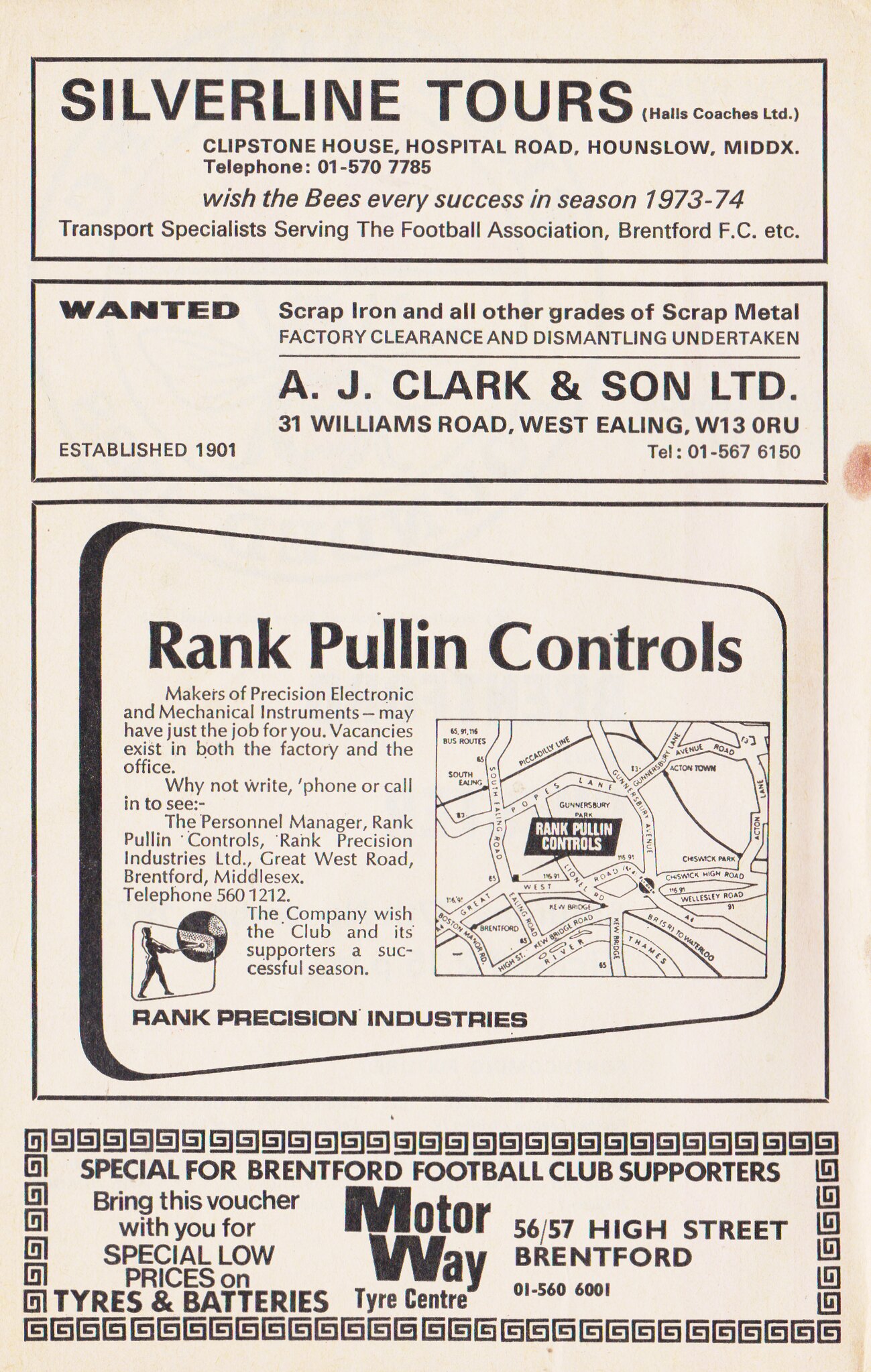This detailed image appears to be a page from either a magazine or a newspaper, exclusively showcasing a series of black and white advertisements. The layout consists of four distinct advertisements stacked vertically, each promoting different businesses and offerings. At the very top, there's an advertisement for "Silver Line Tours," which includes additional details such as "Clipstone House Hospital Road, Middlesex," and a phone number "01-570-7785." This ad wishes the Brentford Football Club, known as "the Bees," success in the 1973-74 season and mentions the company as a transport specialist serving the Football Association.

Immediately below, there's an advertisement from "A.J. Clark and Son Limited," highlighting services related to scrap iron and various grades of scrap metal. The next segment features "Rank Pull-in Controls," associated with "Rank Precision Industries," and accompanied by a small map.

At the bottom, there's a special offer for Brentford Football Club supporters from the "Motorway Tire Center," which advises bringing in a voucher for special low prices on tires and batteries. The entire page is in shades of tan, black, and white, giving it a vintage and utilitarian aesthetic.